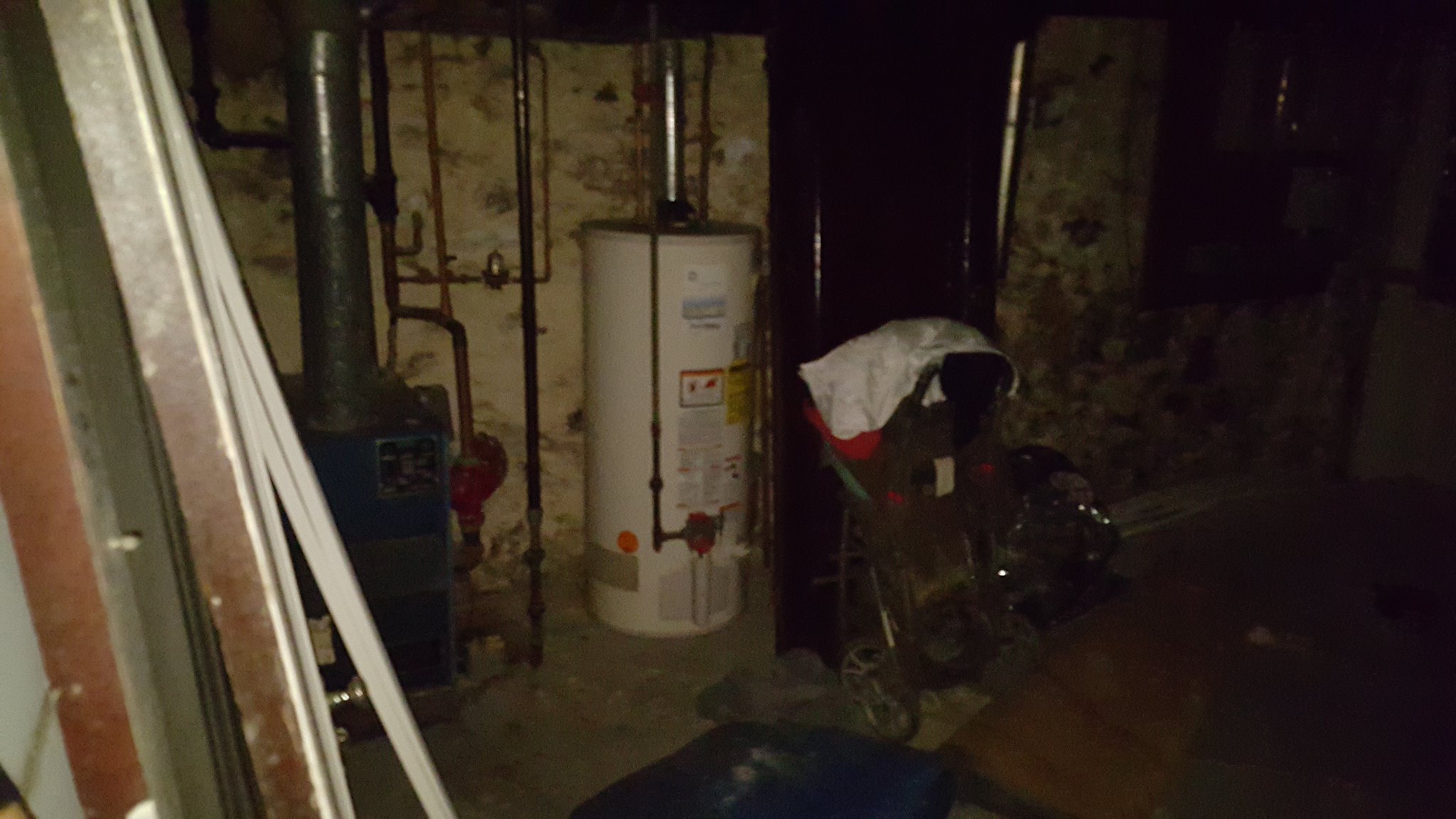The photograph depicts an unfinished, unpainted basement with marked and blemished pale walls. Central to the image is a large, white cylindrical water heater with instructional labels adhered to its surface. Copper and silver pipes extend from the heater, contributing to the cluttered appearance. To the left of the water heater stands a furnace with a square blue base and a large, round metal vent protruding from its top. Adjacent to the heater, an old abandoned baby stroller with a white towel draped over it can be seen. Scattered around the floor are miscellaneous items, including blue objects, small red and silver pipes, and stacked pieces of wood painted white and brown. The overall scene is dimly lit, emphasizing the neglected and disorganized state of the basement.